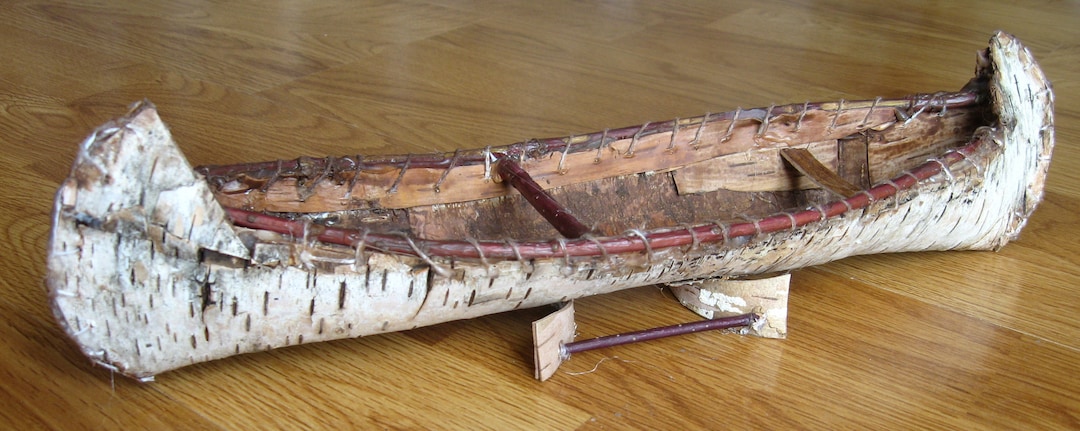The image depicts a handmade model of a birchbark canoe placed on a hardwood floor, illuminated by the soft light that highlights its intricate details. The canoe is constructed from authentic birchbark, with the characteristic white exterior marked by dark lines, reminiscent of traditional Native American canoes from the 1600s. The birchbark is stitched to the ribs of the canoe with visible thread slightly thicker than sewing thread, reinforcing its handcrafted nature. The reddish wood sides and interior planks not only provide structural support but also a contrast to the birchbark. The canoe features a crossbeam and a small bench seat towards the lower right-hand side, showcasing meticulous attention to details. It is mounted on a handmade wooden stand, elevating it slightly off the floor, which draws attention to its crescent-shaped prow and stern. Despite being a model, this canoe's rough interior and functional elements signify a labor of love and skill, faithfully replicating historical canoe designs.